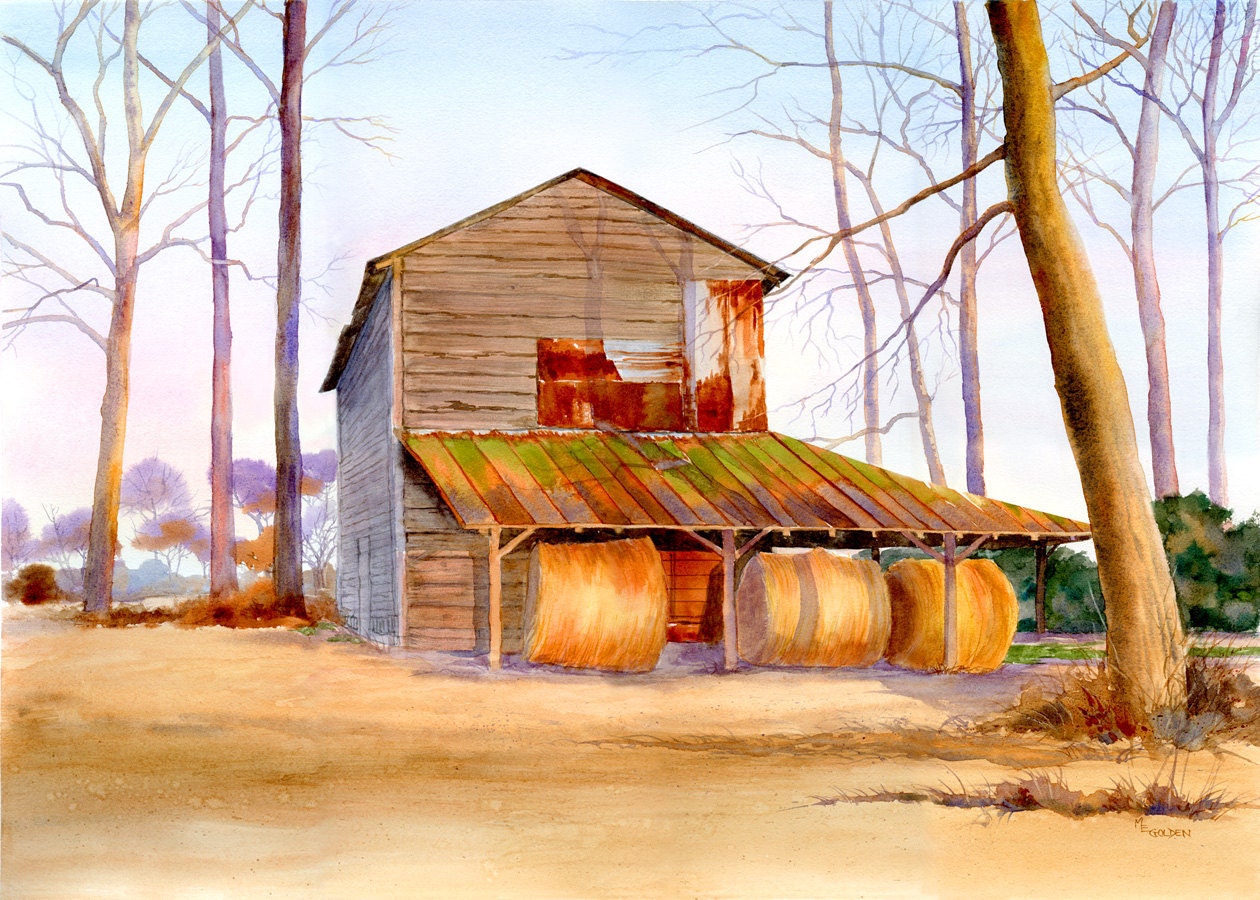An illustration-style image depicts a side view of an old wooden house with a green, weathered roof overhang. The dilapidated structure shows significant damage, rendering parts of it translucent, allowing a glimpse through the house. Beneath the overhang at the front, tree branches are visible. The foreground features hay bales scattered over tan-colored dirt. Surrounding the property are barren, leafless trees, while the background showcases watercolor-style trees adorned with orangey foliage and leaf piles. On one side of the scene, green bushes add contrast to the desolate appearance. The blue sky overhead completes the backdrop of this evocative depiction of neglect and nature's encroachment.